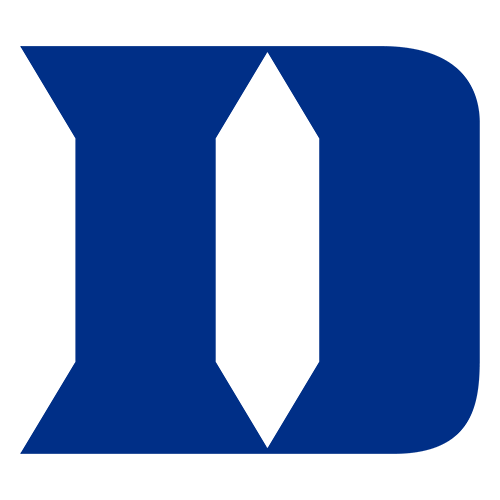The image features a striking blue and white representation, predominantly showcasing a stylized 'D.' The 'D' appears to be inspired by Greek or Roman script, giving it an ancient, geometric elegance. 

In the middle of the 'D,' there is an intricate white cut-out divided into three main segments: a diamond at the top, a slender rectangular bar in the middle, and another diamond at the bottom. This white cut-out creates an illusion of depth and complexity within the blue 'D.'

The 'D' itself has distinct characteristics. The right-hand side of the 'D' is rounded, creating a smooth, continuous curve. In contrast, the left-hand side is more angular and structured, resembling a capital 'I' with slanted triangles at both the top and the bottom. The entire design is centered and exudes a sense of symmetry and balance.

The blue used in the 'D' is a dark navy hue, contributing to the image's bold and authoritative aesthetic. The combination of geometric shapes and the precise use of color make this a visually compelling and unique portrayal of the letter 'D' in a conceptual context.